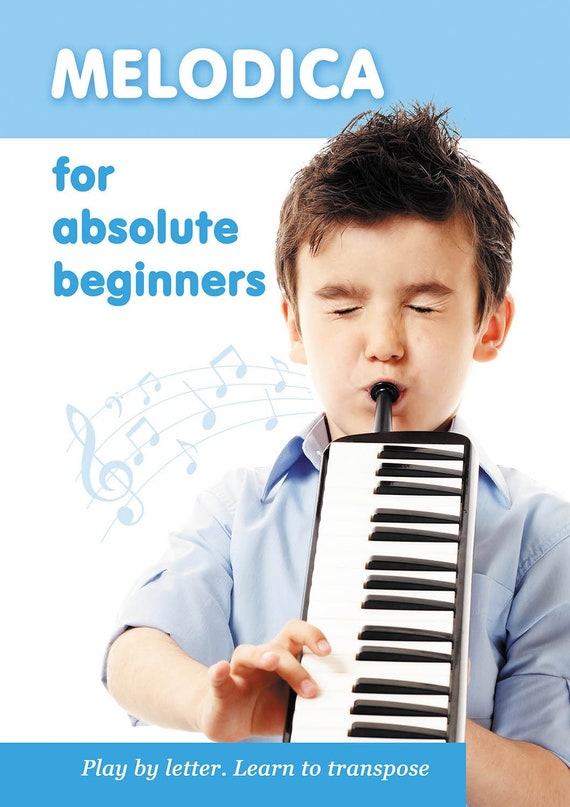This image is an advertisement promoting a melodica for children. The top of the image features a light blue banner with bold white capital letters that read "MELODICA." Below that, on a white background, larger blue text states "FOR ABSOLUTE BEGINNERS." Central to the image, a young boy, around 10 years old, with dark brown hair and wearing a blue polo shirt, is shown playing the melodica—a unique instrument that combines a horn with keyboard keys. The boy's eyes are closed as he blows into the melodica and places his fingers on the keyboard. An illustration of musical notes emanates from the melodica, emphasizing its musical focus. At the bottom of the image, a darker blue box with white text encourages with the phrases "Play by Letter, Learn to Transpose." This advertisement effectively highlights the melodica as an ideal instrument for young beginners looking to learn music.